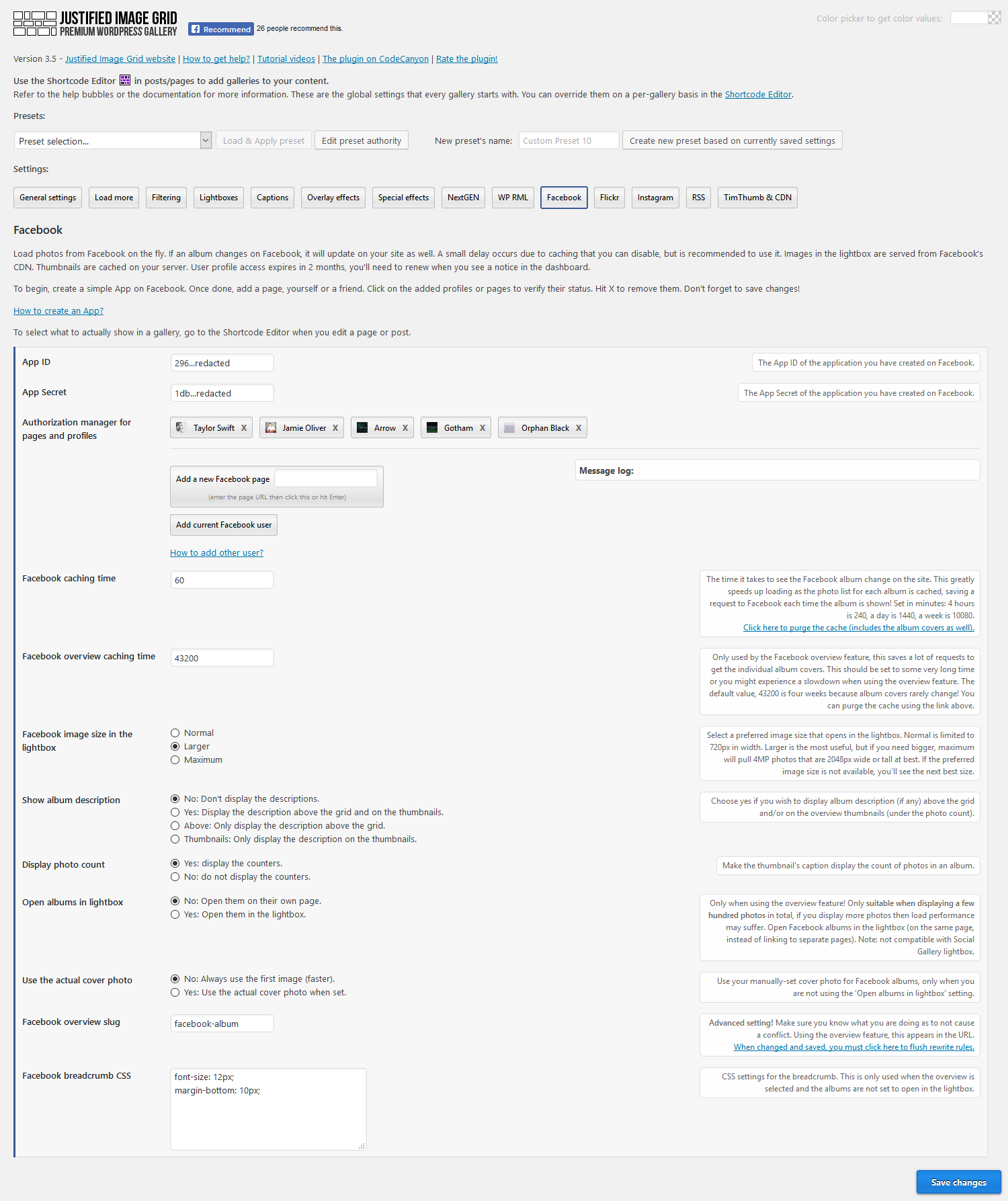### Detailed Descriptive Caption:

This image is a cropped and minimized screenshot of a website page with various elements organized in a compact layout due to its reduced size. The page has a uniform gray background. 

At the top left corner, there is a small, black-and-white logo featuring a segment of a brick fence. Directly to the right of this logo, in black and bold lettering, are the words "Justified Image Grid, Premium Gallery." 

Adjacent to the logo towards the right, there is a blue bar intended for Facebook login. Further right, the site features five categories displayed in a very small gray font. To the right of these categories is a diminutive search box.

Beneath the logo and the header text, blue text is present, although it is difficult to decipher due to the minimized view. Below this blue text are seven text boxes arranged horizontally across the top section of the page. The first of these text boxes includes a 'Go' button on its right. 

Continuing below these elements, there are 14 categories listed horizontally, extending across the page's top section. On the far right of this section, one button is highlighted or selected. Below this, on the left side, the word "Facebook" is visible with a couple of paragraphs underneath.

Towards the center and bottom of the page, on the left side, there are settings menus. To the right of these settings, multiple text boxes, drop-down menus, and selection bubbles are arranged vertically down the screen. Adjacent to these elements, a large white box contains text formatted in paragraphs. In the bottom right corner of this white box, there is a conspicuous blue button that provides options to either save or continue.